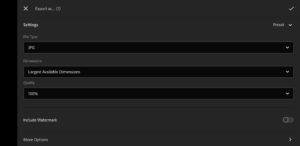This image is a screen capture of a user interface menu from a website or computer program, featuring a predominantly black background. On the far left edge of the image, there is a vertical bar with a deep black color. The central focus of the capture is an exceedingly small menu, making the text illegible. This primary menu has a slightly off-black hue, leaning towards a very dark gray.

In the upper left corner of this menu, there is a distinct "X" icon, accompanied by some faint, unreadable text, suggesting that this icon is likely for closing the menu. On the top right corner, a checkmark icon is present, with an indiscernible word beneath it, and an arrow that implies the presence of a drop-down menu. Adjacent to these icons are more text elements that are also too small to decipher.

Below these elements, the interface features three horizontal menu bars. These bars appear interactive, suggesting that users can click on them to reveal additional options. Further down, there is more white text, adding to the information density of the menu. On the far right, there seems to be a gear icon, typically indicative of settings, but its small size makes it hard to confirm its exact purpose. The overall interface is compact and text-heavy, with many elements too small to clearly identify.